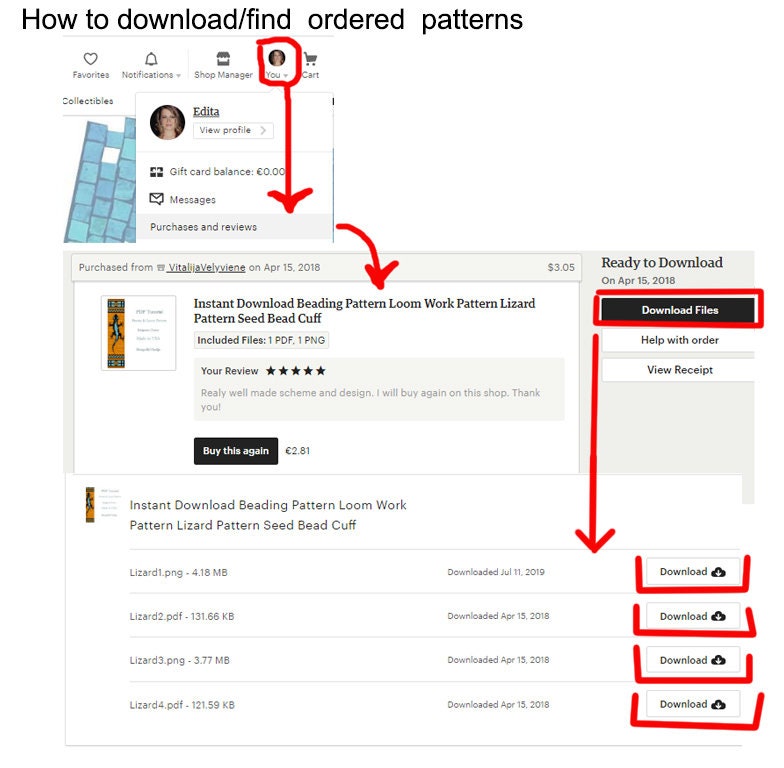Title: "How to Download/Find Ordered Patterns"

Description:
The image showcases a tutorial screen with comprehensive visual instructions on downloading and finding ordered patterns. At the very top of the screen, black text reads, "How to Download/Find Ordered Patterns." 

The main section of the screen features a light gray ribbon spanning the top. A prominent red arrow points to a specific product for sale, titled “Instant Download Beading Pattern, Loom Work Pattern, Lizard Patterns Cuff." 

Above this product, there is a small pop-up box that includes a user profile photo labeled "User's Name." This profile photo is circled in red, with an arrow directing viewers to the section labeled "Purchases and Reviews," which is highlighted.

Several red arrows and circles are distributed across the page to emphasize important elements. Every available download option is clearly highlighted in red. One notable highlight is the “Download Files” button, which is outlined with a red border and has an arrow pointing downwards to indicate all downloadable files.

The detailed red annotations throughout the screen guide the user step-by-step, ensuring clarity on where to find and how to access the ordered patterns.